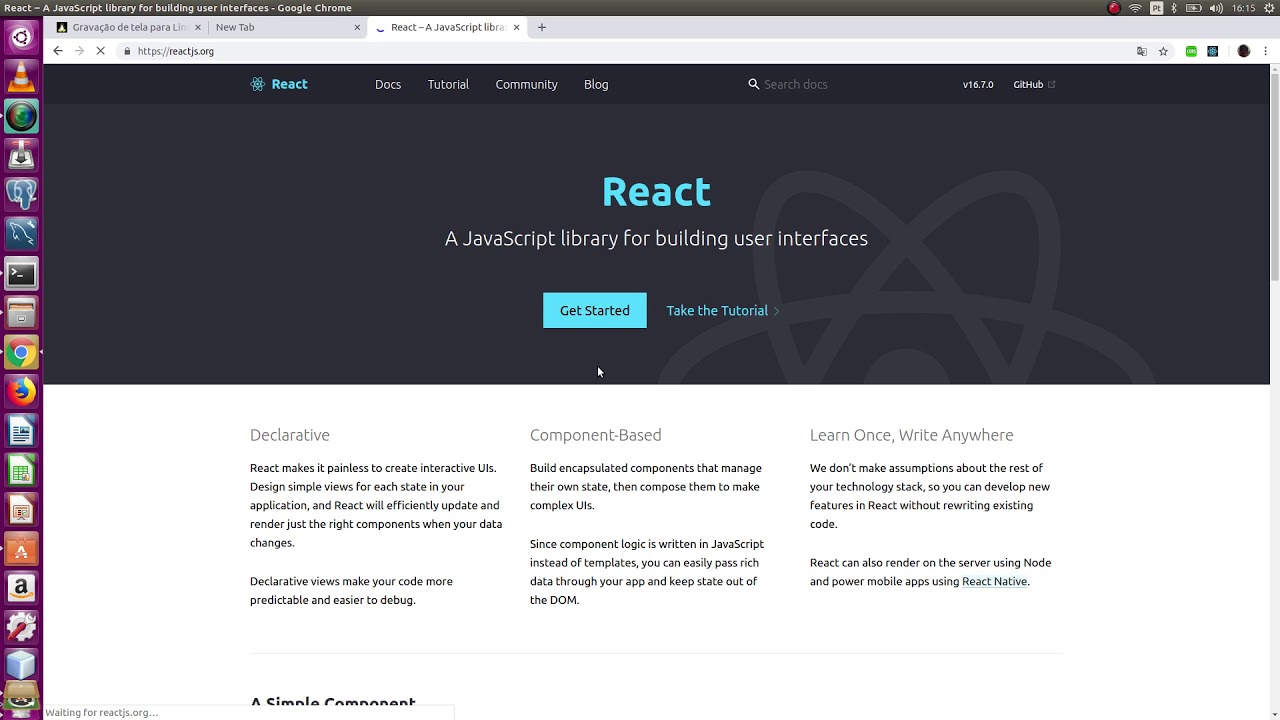This is a detailed screenshot of a homepage of the official React website taken on Google Chrome. At the top left of the browser, there are three open tabs. The current tab is labeled "React - A JavaScript library," while the tab on the left shows Portuguese text: "Gravação da Tela para a Lenda."

On the left-hand side of the screen, there's a tall vertical purple sidebar featuring a variety of icons. The recognizable icons include an orange traffic cone (VLC media player), an elephant (likely representing PostgreSQL or PHP), a blue square with a dolphin (MariaDB or MySQL), the Google Chrome logo, Mozilla Firefox, Microsoft Word, Microsoft Excel, Amazon, and possibly a Linux icon, among others.

In the top left-hand corner of the browser window, it reads "React - A JavaScript library for building user interfaces | Google Chrome." Below this, there is a black navigation menu bar with links labeled React, Docs, Tutorial, Community, and Blog, along with a search input field. The URL in the address bar is "https://reactjs.org".

The screenshot was captured at 16:15. The main content of the web page features a gray section with an atom-like design and blue text that reads "React." Beneath this, the tagline "A JavaScript library for building user interfaces" is displayed, and there is a prominent blue button labeled "Get Started" next to blue text that says "Take the Tutorial."

At the bottom part of the screenshot, there are three columns with headings: "Declarative," "Component-Based," and "Learn Once, Write Anywhere." These sections likely contain additional information relevant to each heading.